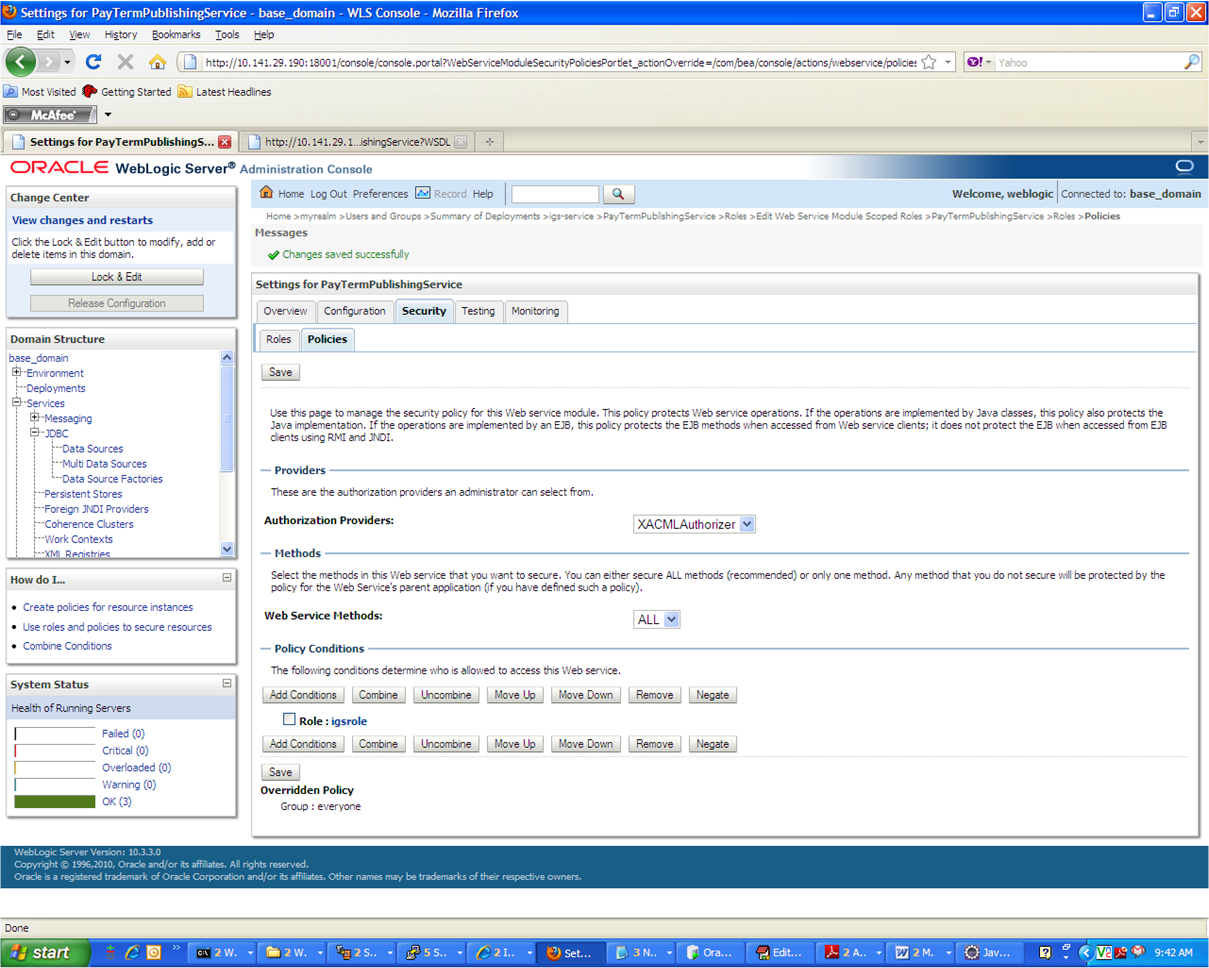This screenshot captures the interface of the Mozilla browser displaying the Oracle WebLogic Server Administration Console with a variety of detailed elements.

At the top, the standard browser features are present: a menu bar, navigation buttons to the left of the address bar, and a bookmarks toolbar featuring "Most Visited," "Getting Started," and "Latest Headlines." Additionally, a small McAfee banner is visible.

There are two open tabs, with the first tab presenting the "Settings for Payterm Publishing Service" webpage. The webpage is divided into two main sections. The left section features a sidebar with four distinct boxes and the header "Oracle WebLogic Server Administration Console" in red, all caps text. The boxes in the sidebar include:

1. **Change Center**:
   - Contains two buttons: "Lock & Edit" and a grayed-out "Release Configuration."

2. **Domain Structure**:
   - Displays a tree-like structure that can be expanded.

3. **How Do I**:
   - Lists three bullet points.

4. **System Status**:
   - Features a bar graph illustrating the health of running servers, with the "OK" status highlighted by a green bar.

Adjacent to the sidebar, the main section of the webpage has a white background. The header bar includes options such as "Home," "Logout," "Preferences," "Record," and "Help," along with a search bar and search button. Below this, a message section, indicated by a green check mark, confirms that "Changes saved successfully."

Further down, the detailed "Settings for Payterm Publishing Services" section appears. It includes tabs labeled "Security" and "Policies," with an additional save button at the top. The content of this section is organized into three subsections: "Providers," "Method," "Web Services Method," and "Override Policy."

The entire layout is designed for easy navigation and management, catering specifically to administrative tasks in Oracle WebLogic Server.